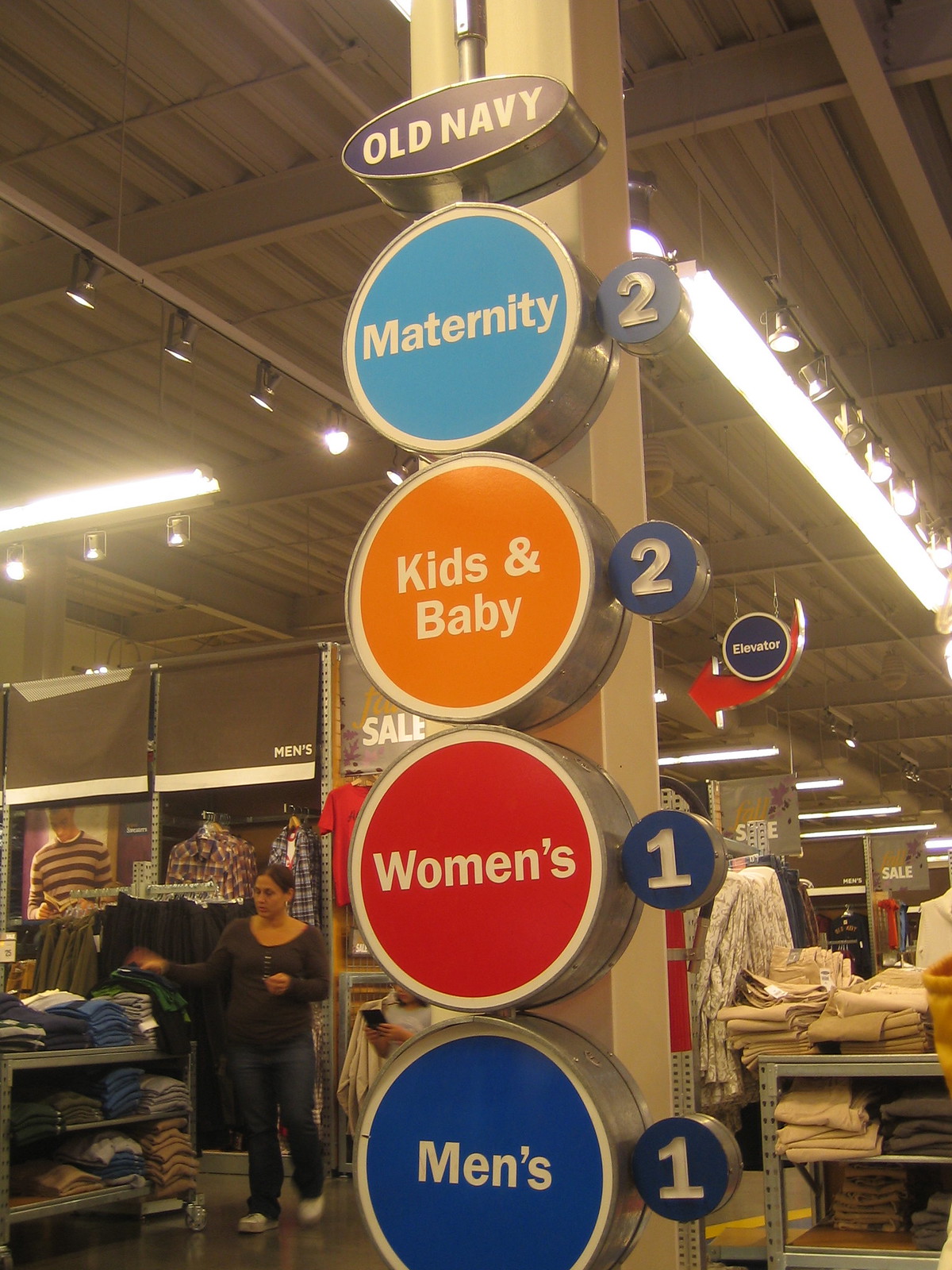The photograph captures the interior of an Old Navy store, characterized by its warehouse-like structure with a high corrugated metal roof and suspended spotlights. Dominating the center is a tall, tan-colored steel column adorned with a series of distinct, colorful circular signs indicating different departments. At the top of the column, a dark oval sign with tan lettering prominently displays the store name "Old Navy." Directly beneath it, a round sign with white trim for the "maternity" section followed by a yellow circle for "kids and baby," a red circle for "women's," and a blue circle for "men's." Each section sign is accompanied by a smaller dark circle, indicating either the number one or two, designating specific areas within the store. The surrounding area features neatly organized tables filled with folded jeans and shirts. To the left, a woman with dark hair pulled back into a ponytail, dressed in a dark shirt, blue jeans, and white sneakers, is seen placing a pair of jeans onto a table, adding to the well-organized display of clothing.